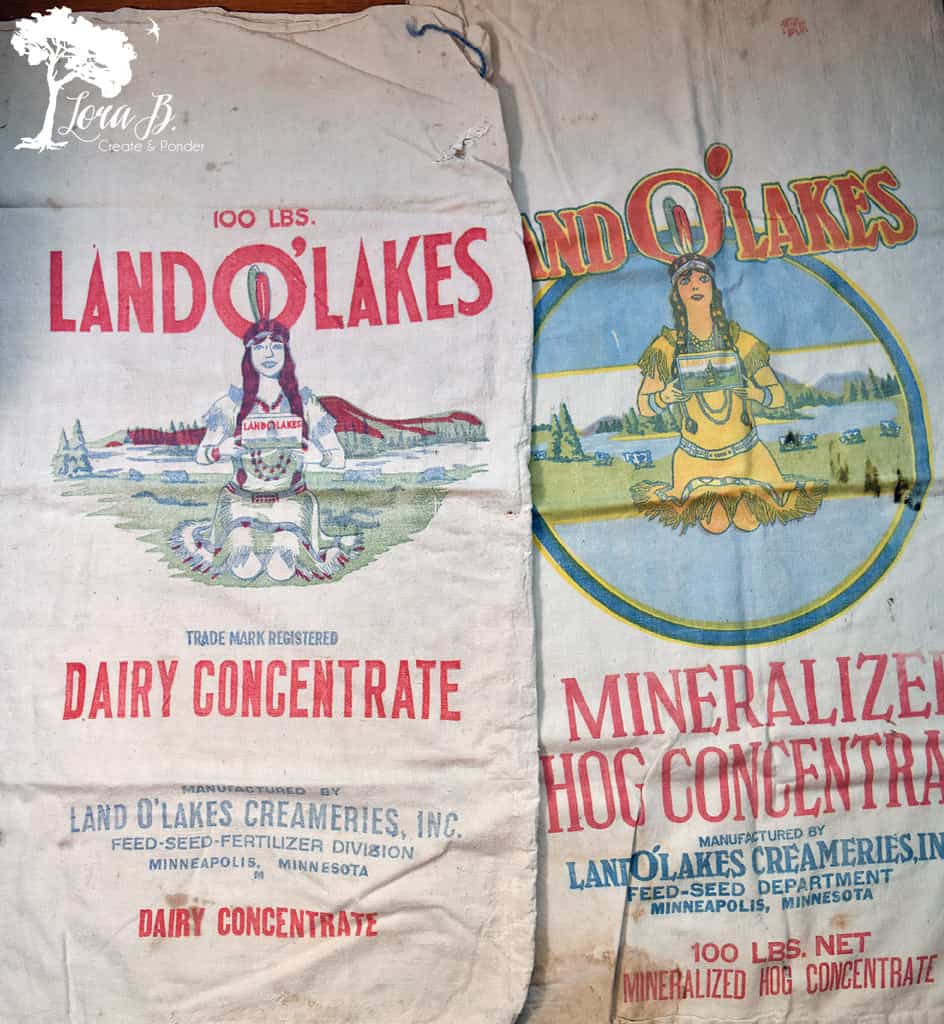This image displays two burlap bags featuring vintage Land O'Lakes packaging. On the left is a slightly off-white bag labeled "100 Pounds Land O'Lakes Dairy Concentrate," showcasing the retired logo of a Native American woman kneeling and holding a box. The text includes "Trademark Registered" and "Manufactured by Land O'Lakes Creameries, Inc., Feed Seed Fertilizer Division, Minneapolis, Minnesota," with "Dairy Concentrate" reiterated in red. The bag to the right, similarly adorned, reads "Land O'Lakes Mineralized Hog Concentrate" and includes "100 Pounds Net, Mineralized Hog Concentrate," also manufactured by Land O'Lakes Creameries but specified as the Feed Seed Department. Both bags feature similar design elements, colors, and the depiction of the Native American woman, with detailed descriptions of her traditional attire and jewelry, including long dark hair, beaded jewelry, and feathers. In the upper left corner of the image is a white logo of a tree with the inscription "Laura B. Create and Ponder."